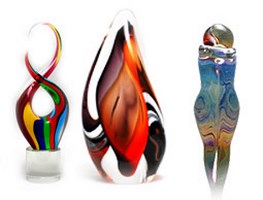This image showcases three distinctive blown glass sculptures, each uniquely colorful and intricately designed. The first sculpture, placed on a small white marble square, is shaped like a figure eight with varying thickness. It displays a vivid array of colors: red at the top of its loop, followed by yellow, black, green, red, and light blue descending in sequence. The second, more prominent sculpture, resembles a teardrop or an egg, featuring black and white rims with a vibrant mix of purples, light reds, and darker reds in the center. The third sculpture presents an imaginative form that seems to resemble a female torso or a tooth with two roots; it has a silver marble perched on top. This piece transitions from swirly blue at the top through tan hues, finishing with blue again at the two leg-like roots. Each sculpture exhibits curvy, swirly designs and melds of colors, contributing to their abstract and decorative appearance.